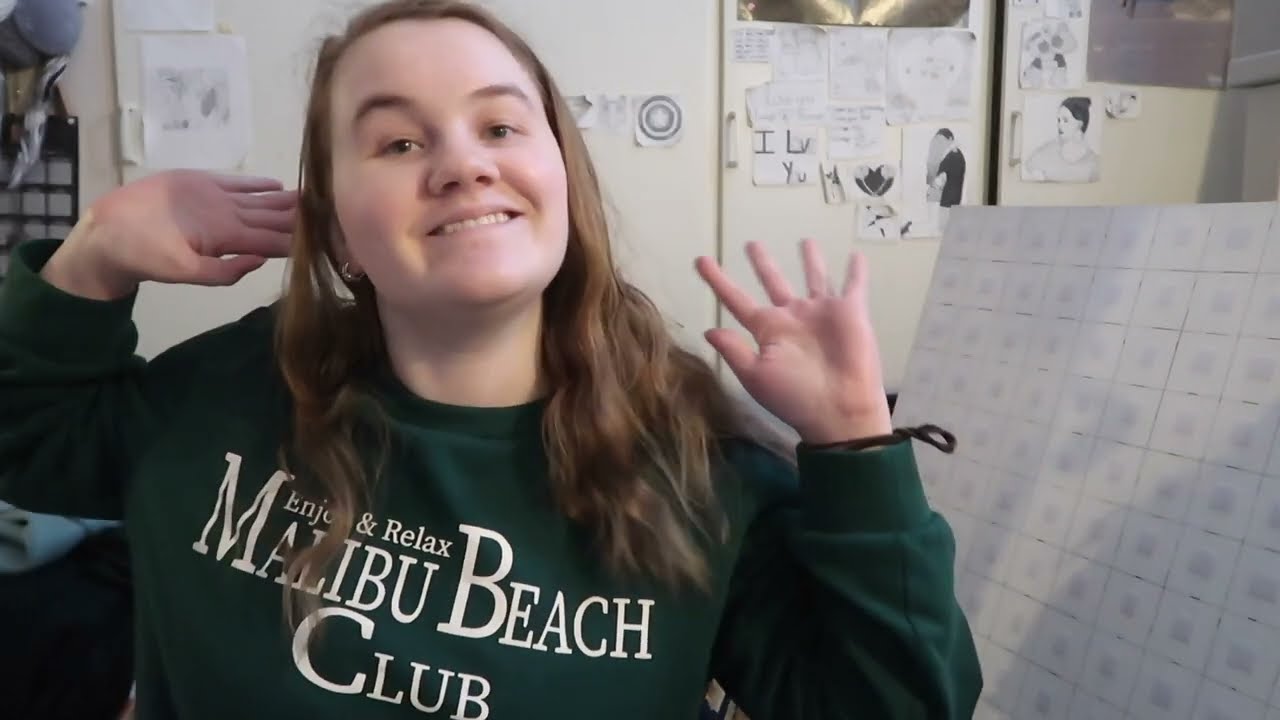The horizontal, rectangular image features a young Caucasian woman posing for the camera in what appears to be an art studio or classroom. She is positioned from the left side to the center, with a focus on her upper body from the chest up. The woman has long brown hair parted on one side, cascading down to her chest. She is wearing a dark green sweatshirt with white text that reads, "Enjoy and Relax Malibu Beach Club." Her arms are raised with elbows bent, displaying her open palms facing outward and fingers visible. She is smiling slightly, though it appears she is biting her bottom lip with only her top teeth showing, giving her lips a thin appearance. Behind her, the white room's walls are adorned with numerous white papers featuring black pencil drawings, as well as a large whiteboard with black lines. To the far right, a grid board is visible, segmented into many small squares, some of which have tape pieces on them. Additionally, scattered artwork and a couple of blue balloons can be seen in the background. The detailed setting and her cheerful yet quirky gesture combine to create an engaging and vibrant scene.